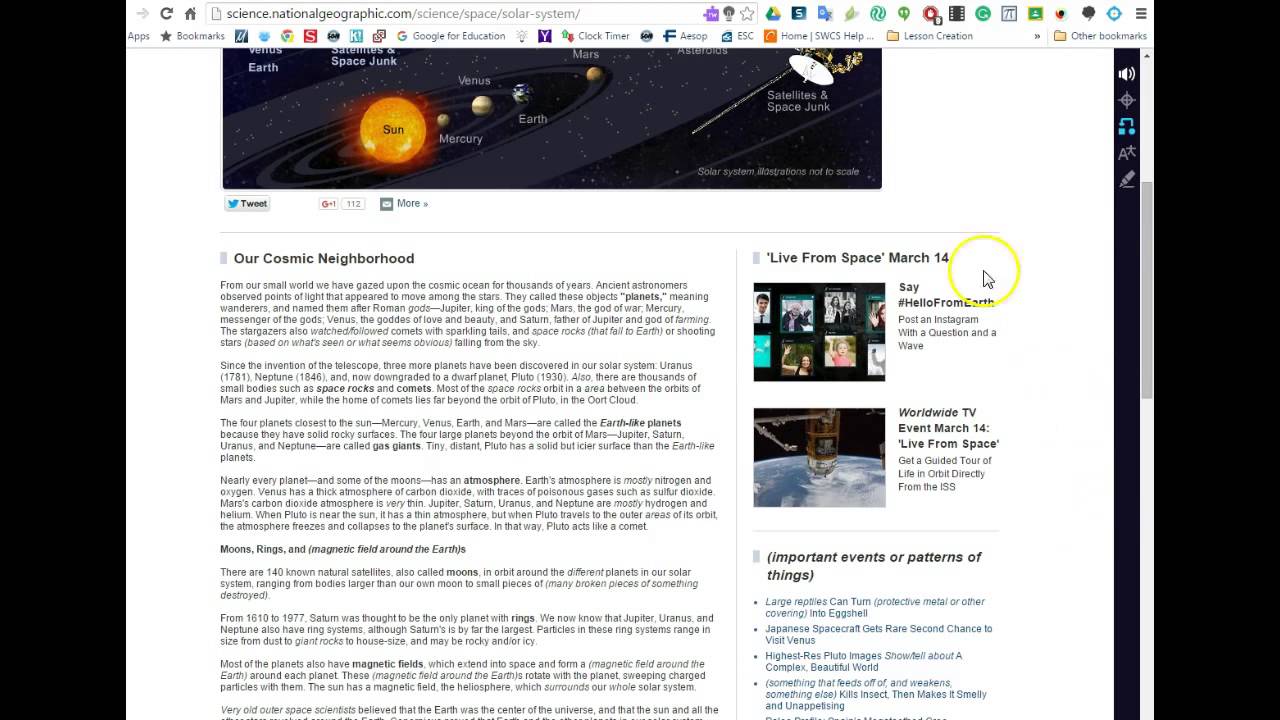This narrative describes a detailed screenshot of a webpage from National Geographic's science magazine on their website. 

**Caption:**

A detailed screenshot of the National Geographic science magazine webpage captures a comprehensive overview of our solar system and its components. At the top lies the web browser header with the URL: science.nationalgeographic.com/science/space/solar-system/. The header is adorned with various functional icons. Immediately beneath, the webpage features a vivid diagram of the solar system. The Sun is positioned in the lower left corner, while the planets trail upward and to the right. A satellite labeled "Satellites and Space Junk" also appears on the right side of the image. The illustration is annotated as "Solar system illustrations not to scale" in the bottom right corner.

Further down, interactive buttons are displayed against the white background: a tweet button in the bottom left, a Google Plus button indicating "112," and an email button labeled "more." A thin gray line demarcates the header from the article below. 

The left section of the page presents an article titled "Our Cosmic Neighborhood," accompanied by several paragraphs. The introductory text reads: "From our small world, we have gazed upon the cosmic ocean for thousands of years. Ancient astronomers observed points of light that appeared to move among the stars. They called these objects planets, meaning wanderers, and named them after Roman gods: Jupiter, king of the gods; Mars, the god of war; Mercury, the messenger of the gods; Venus, the goddess of love and beauty; and Saturn, father of Jupiter and god of farming. Stargazers also followed comets with sparkling tails and witnessed space rocks falling to Earth, known as shooting stars, from the sky."

The layout and content provide an educational and visually appealing resource for understanding our solar system and its history observed from Earth.